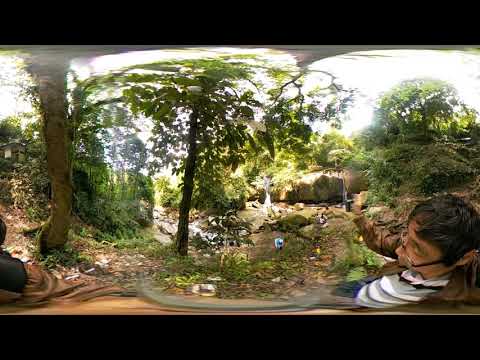This distorted and blurry outdoor photo appears to be captured using a virtual reality lens, contributing to its warped appearance. Set in a lush, green forest, the image prominently features a man with brown hair and clear plastic-framed glasses. He can be seen in the lower right-hand corner, dressed in a white, gray, and black t-shirt under a brown jacket, with blue pants. The man seems to be taking a selfie with a selfie stick while following another individual dressed in tan pants and a black and tan jacket. The forest backdrop includes numerous trees and plants, with leaves scattered on the ground and a small creek bordered by rocks. The sky is partially visible, adding to the outdoor ambiance. Black rectangles frame the top and bottom of the image, indicating possible digital manipulation or framing.